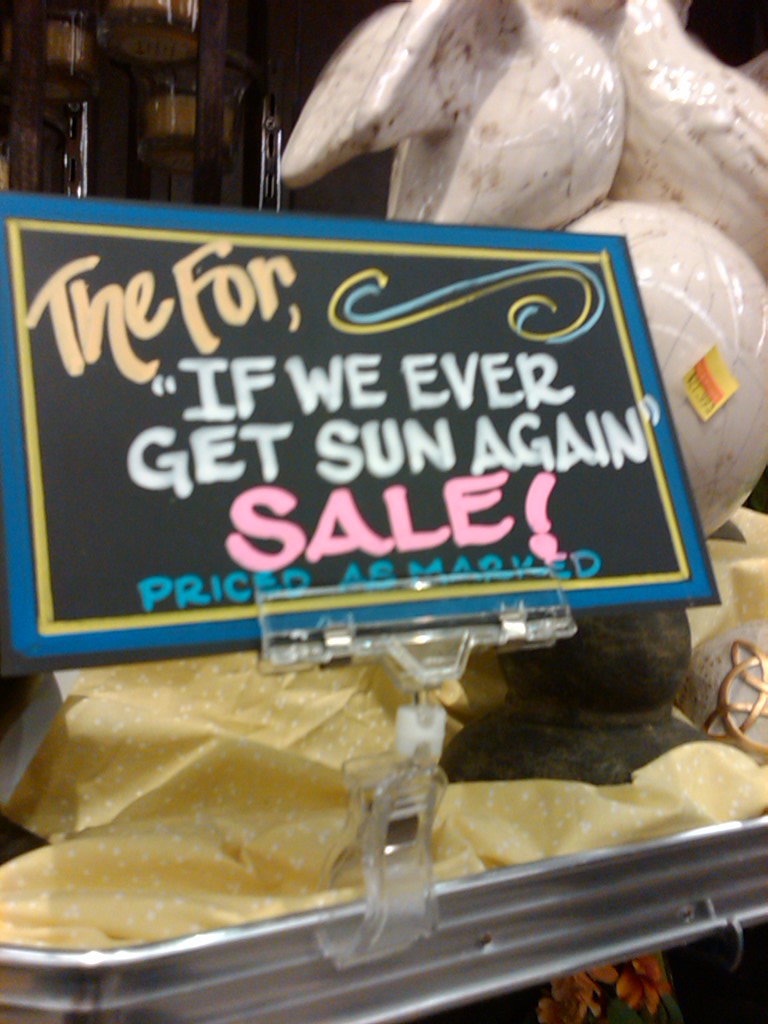Photograph in a store featuring a hand-made sale sign. The sign displays the text "If we ever get sun again" in sarcastic quotation marks, followed by "SALE!" and "Price as marked." The lettering is color-coded: "SALE!" is in vibrant pink, "Price as marked" is in calming blue, "If we ever get sun again" is in crisp white, and the numeral "4" is highlighted in bright yellow for emphasis. The background reveals a hint of the store's merchandise, including a visible yellow price tag on an unidentified object, further accentuating the casual and cheerful ambiance of the store.